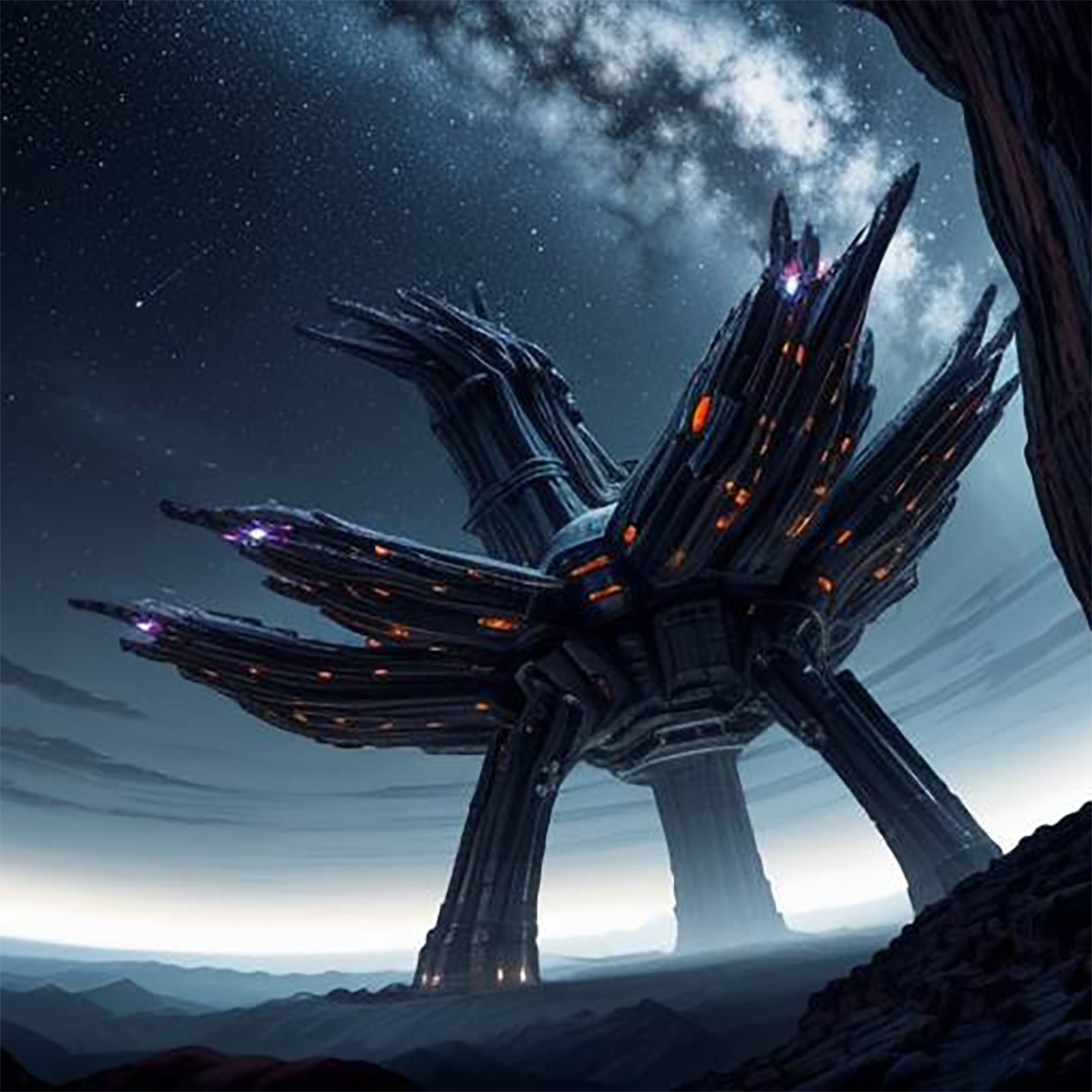The image depicts a dark gray, potentially CG-rendered or drawn, colossal structure that could be a spaceship or a robot, evoking a foreboding and daunting presence. The structure resembles a tripod with three enormous legs converging to support a large disk at the top. From this disk, several arm-like structures jut outwards, resembling the ripped ends of highways, with a towering central arm reaching skyward. The structure is illuminated with vibrant purple, orange, and yellow lights, contrasting starkly with the otherwise neutral tones.

It stands amidst a desolate, mountainous gray rocky landscape, with a navy blue to charcoal black sky above, adorned with numerous white stars and planets, including a dense cluster mimicking an intense view of the Milky Way. Wisps of dark clouds and smoke add to the ominous atmosphere. The sky's illumination, reminiscent of the last light of a missed sunset, enhances the eerie setting. There are no signs of activity or life, underscoring the scene's isolation and vastness. The overall imagery, with its blend of sci-fi elements and dramatic lighting, paints a haunting and otherworldly tableau.